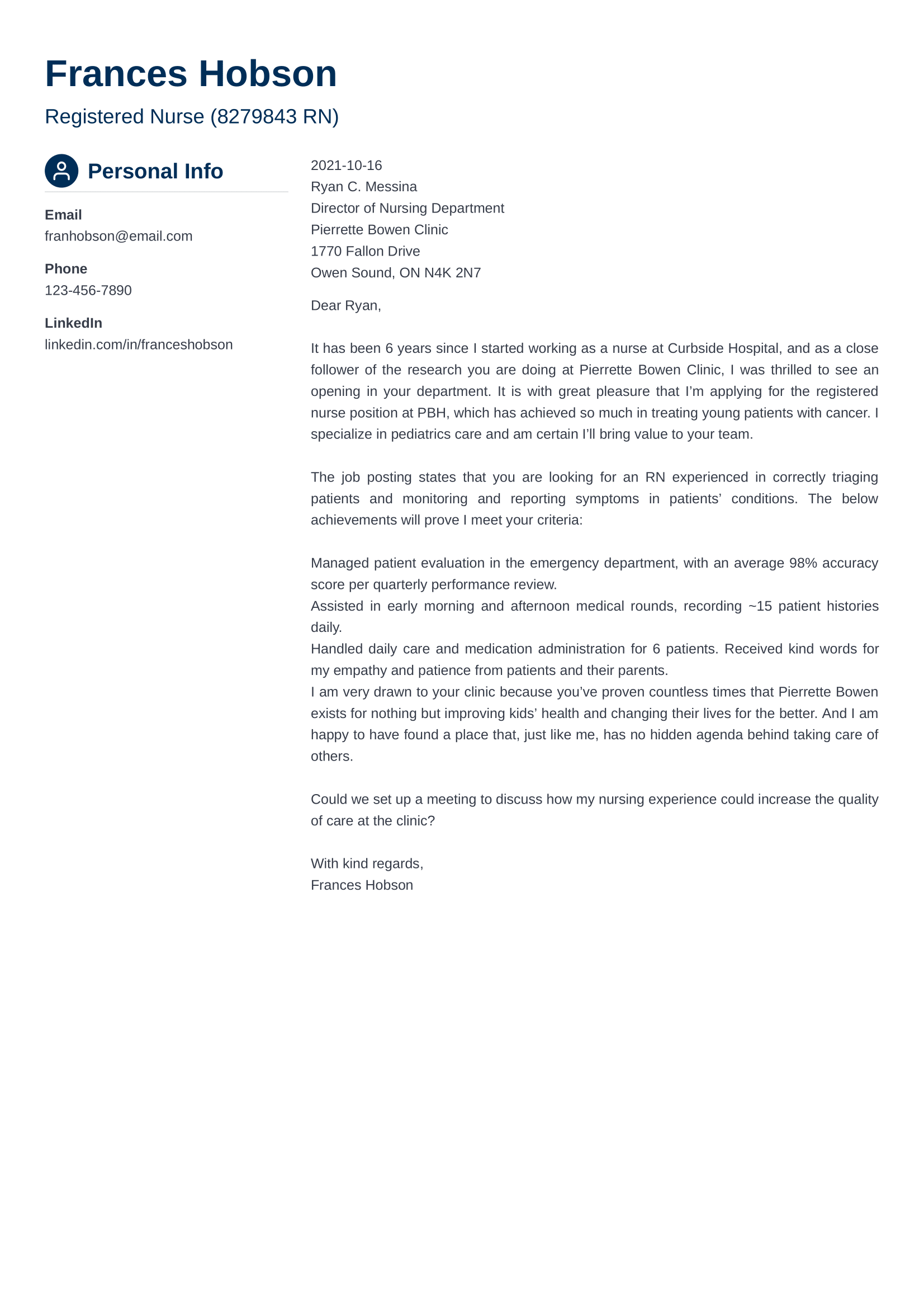#### Caption:
**Frances Hobson - Registered Nurse at Perita Bowen Clinic**

Frances Hobson, R.N. (Nurse Number: 8279843RN) has been a dedicated registered nurse since October 16, 2021. She is currently employed at the Perita Bowen Clinic, located at 1770 Falcon Drive, Owen Sound, ON N4K 2N7. Under the esteemed leadership of Brian C. Messina, the Director of the Nursing Department, Frances has consistently showcased her excellence in pediatric care, particularly in treating young cancer patients.

With a specialization in pediatric care, Frances is passionate about her work and continuously contributes to advancements in young patient care. She has applied for a registered nurse position at PBH, a prestigious institution known for its significant achievements in cancer treatment for young patients.

Frances can be reached via email at franzhobson@email.com or via phone at 123-456-7890. For more about her professional journey, her LinkedIn profile is available at linkedin.com/in/FrancesHobson.

**Background Summary:**
- **Date of Employment:** October 16, 2021
- **Director of Nursing:** Brian C. Messina
- **Current Workplace:** Perita Bowen Clinic, 1770 Falcon Drive, Owen Sound, ON N4K 2N7
- **Contact Information:** 
   - **Email:** franzhobson@email.com
   - **Phone:** 123-456-7890
   - **LinkedIn:** linkedin.com/in/FrancesHobson
- **Specialization:** Pediatric Care, Cancer Treatment for Young Patients

**Achievements & Skills:**
- **Expertise:** Correct patient triaging, symptom monitoring, and detailed reporting of patient conditions.
- **Professional Goal:** To bring her expertise to the team at PBH and contribute to its ongoing success in pediatric oncology.

Frances’ experience and qualifications ensure her capability to excel in this role, promising invaluable contributions to the nursing team and patients alike.